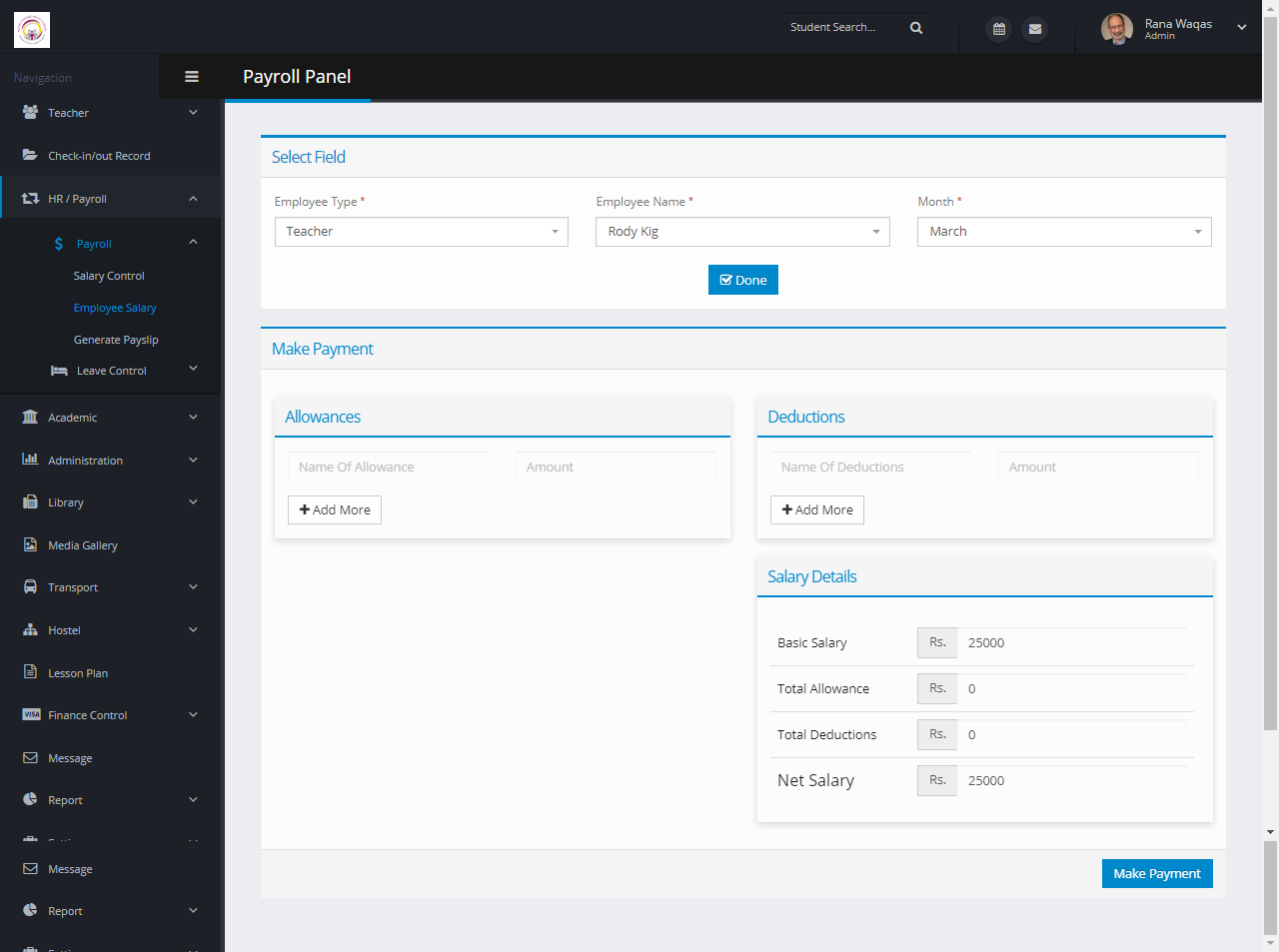**Screenshot of Payroll Page: Detailed Description**

The image is a screenshot of a payroll page within an administrative software interface. 

**Top Right Corner:** 
- A circular profile picture of a man labeled "Grano Vegas Admin" is prominently displayed.

**Left Column:**
- A vertical column showcases various icons paired with explanatory text:
  - **Teacher**
  - **Check In/Out Record**
  - **HR/Payroll**
    - Payroll
    - Salary Control
    - Employee Salary
    - Generate Pay Slip
    - Leave Control
  - **Academic**
  - **Administration**
  - **Library**
  - **Media Gallery**
  - **Transport**
  - **Hostel**
  - **Lesson Plan**
  - **Finance Control**
  - **Message**
  - **Report**

**Main Panel (towards the right side of the page):**
- At the top, the heading "Payroll Panel" is displayed in large print.
  
**Selection Fields:**
  - **Employee Type:** The dropdown menu has "Teacher" selected.
  - **Employee Name:** The dropdown menu has selected "Rody Kig."
  - **Month:** The selected month is March.
  - A blue button labeled "Done" is present beneath these fields.

**Payment Section:**
  - "Make Payment" is the header for this segment.
  - **Allowances Section:** Contains two text boxes:
    - One for the "Name of Allowance."
    - Another for "Amount."
    - There's an "Add More" button below these text boxes.
  - **Deductions Section:** Includes similar text boxes:
    - One for the "Name of Deductions."
    - Another for "Amount."
    - An "Add More" button is below these text boxes.

**Salary Details:**
  - Summarizes:
    - Basic Salary
    - Total Salary
    - Total Deductions
    - Net Salary

**Bottom Right Corner:**
  - A "Make Payment" button is prominently placed.